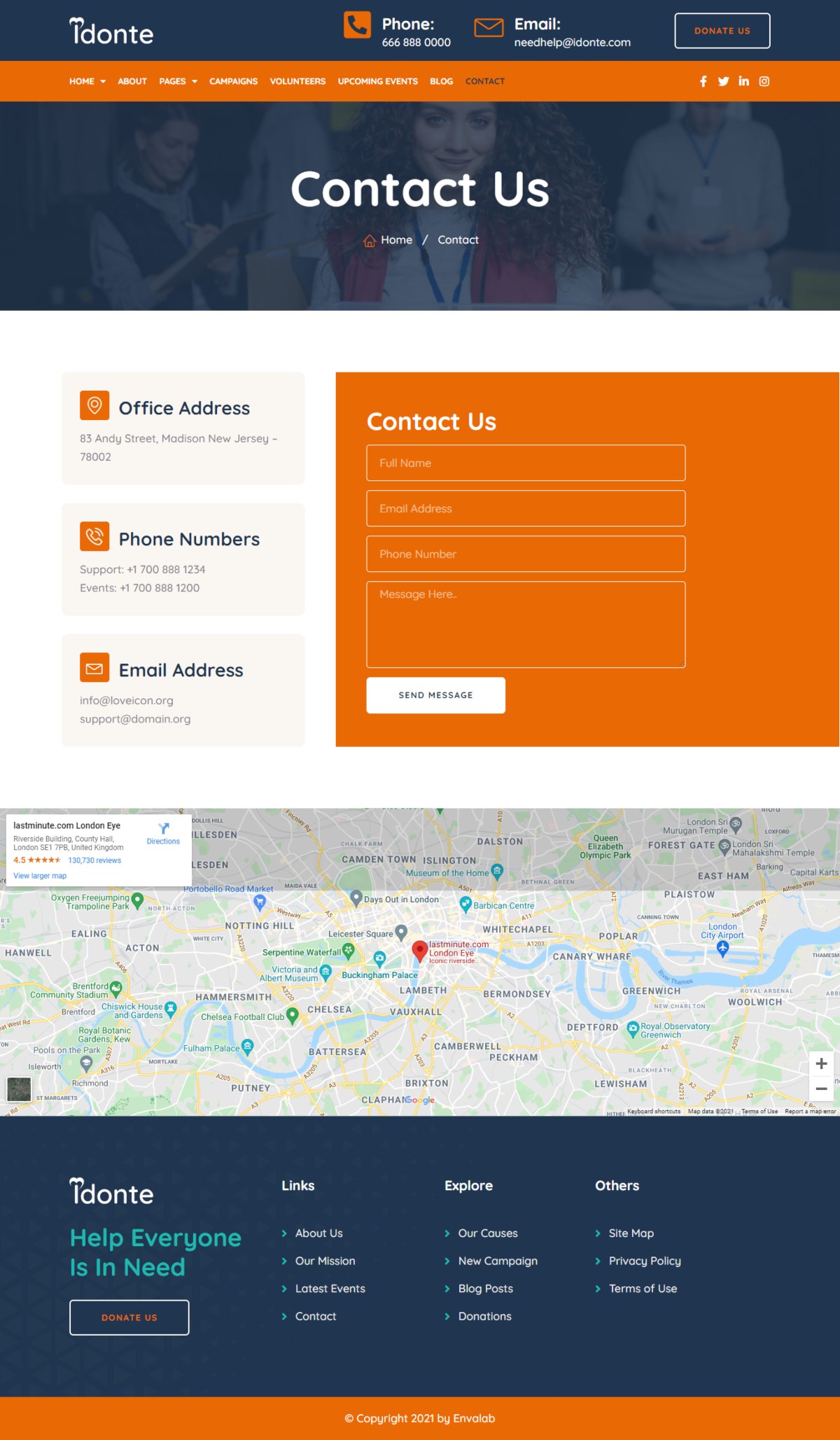The screenshot displays a phone or tablet layout with a predominantly vertical orientation. The design features dark blue backgrounds at both the top and bottom, each highlighted by an orange line. 

At the very top, there's a blue banner with an orange line, and the phrase “Contact Us” is prominently displayed in white letters. The background subtly incorporates the silhouettes of four people.

Below this, the screen is divided into two main sections. The upper section is dedicated to contact information. On the left side, there are three boxes labeled "Office Address," "Phone Number," and "Email Address." Adjacent to these, an orange button labeled “Contact Us” encourages user interaction by providing sections to fill in personal details.

The lower section is occupied by a map spanning the full width of the screen. Though details are small and somewhat indistinguishable, a river and multiple location markers are visible.

Finally, the bottom segment, also with a dark blue background, contains text in white. On the left side, the text "T or I-D-O-N-T" is visible, followed by the phrase “Help Everyone in Need” in turquoise letters. The rest of the bottom section is filled with additional text written in white.